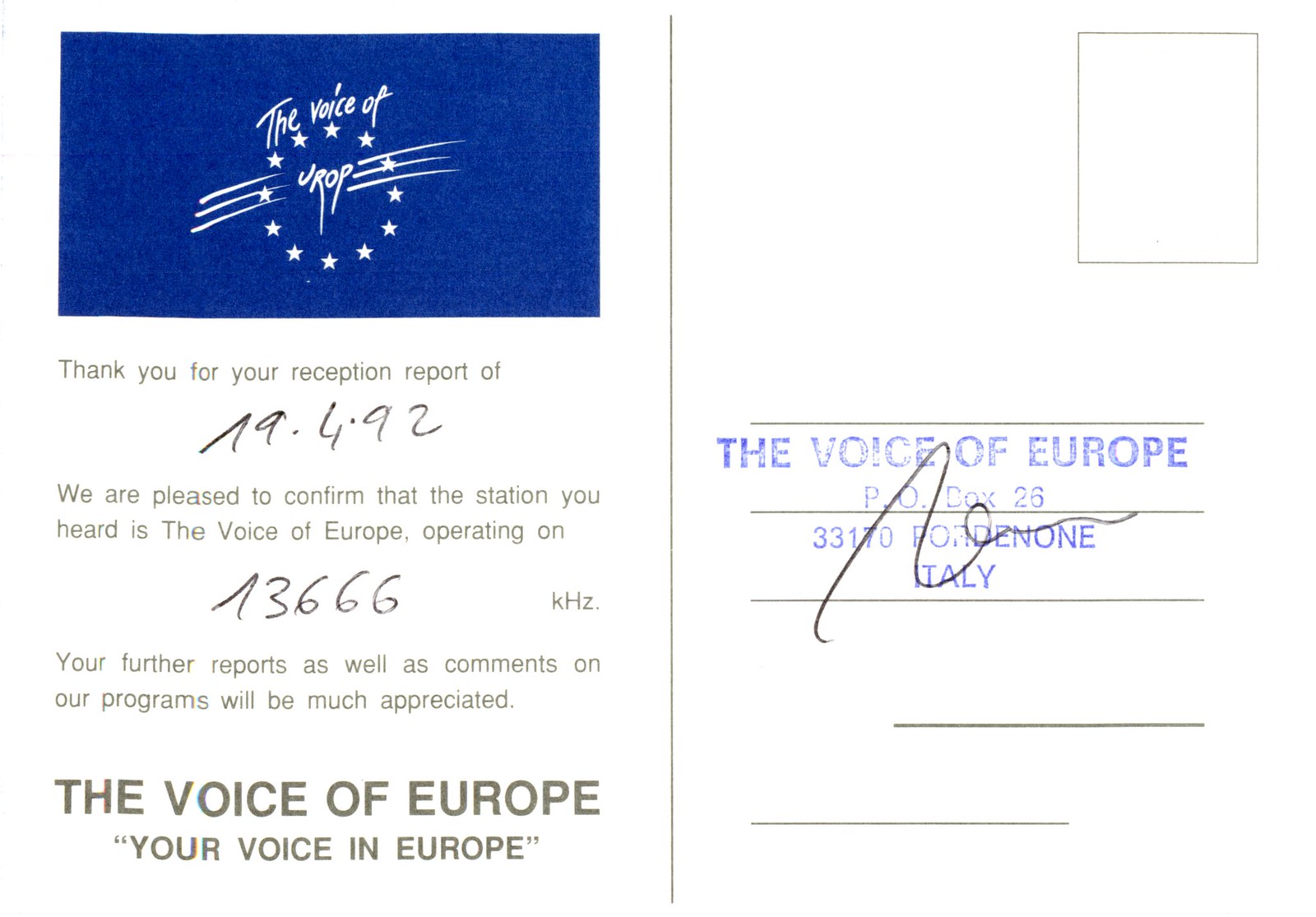The image depicts the back of a postcard from "The Voice of Europe," also spelled "U-RO-P" in their logo. Positioned on the left side of the postcard is a blue rectangular logo featuring a circle made of stars, with the text "The Voice of Europe, U-RO-P" in white font. Below the logo, there's a message thanking the recipient for their reception report of a specific frequency. The message reads, "Thank you for your reception report of A9-4-.92. We are pleased to confirm that the station you heard is The Voice of Europe, operating on A3666KHZ. Your further reports, as well as comments on our programs, will be much appreciated." The logo also includes the tagline "Your voice in Europe" in quotation marks. On the right-hand side of the postcard, there's space designated for an address and a small square in the top right corner for a postage stamp. Additionally, there is a stamped imprint that reads, "The Voice of Europe, P.O. Box 2633170, Portorin, Italy."